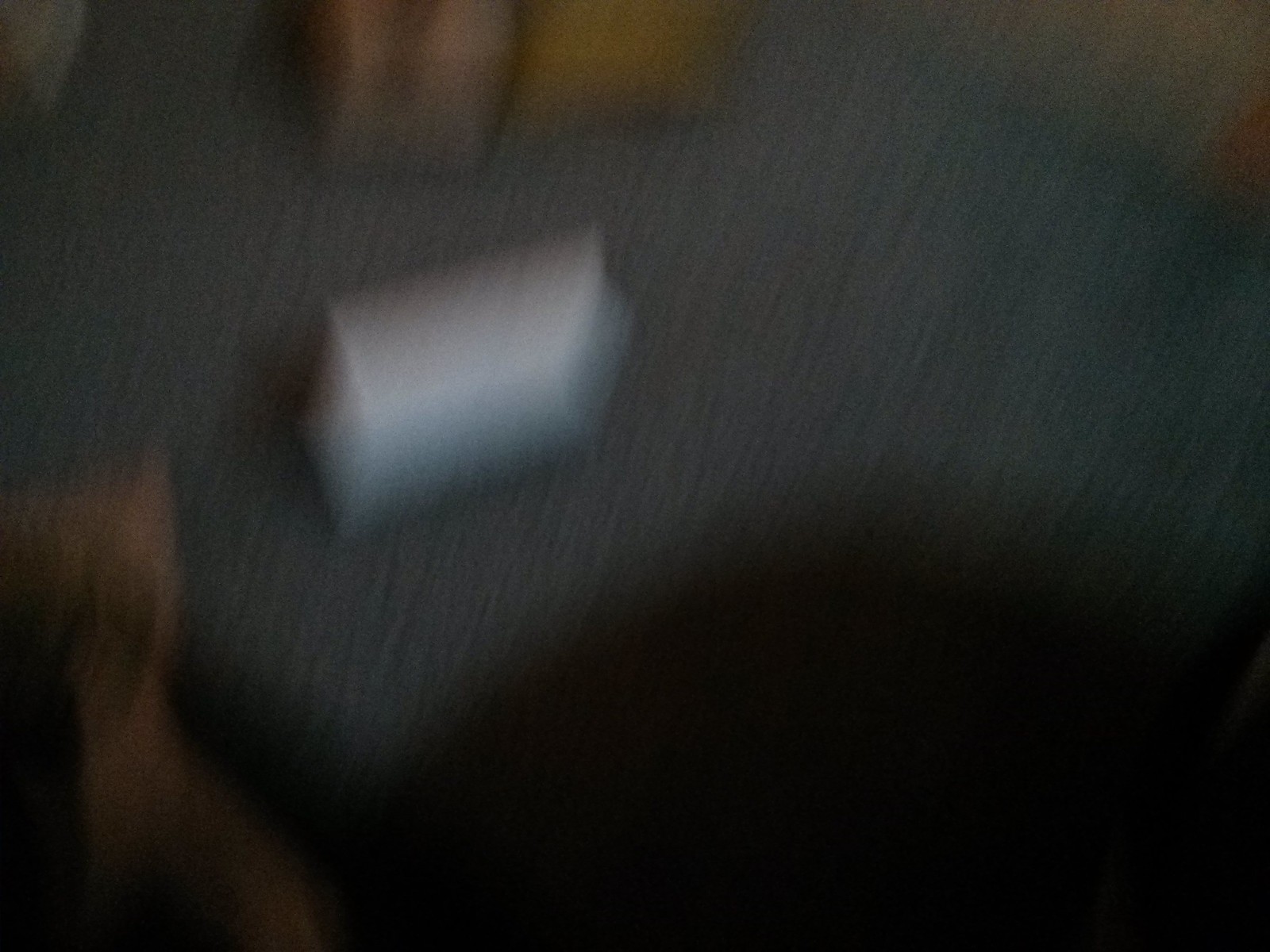This is a very blurry image with indistinct shapes and colors. The bottom portion of the image is predominantly black, with a prominent brown shape originating from the lower left corner and extending to the middle. The central and upper areas of the photo are predominantly dark gray. Within this gray section is a white rectangular shape. In the top left corner, there appears to be a fragment of a cube, possibly brown in color, although it's hard to distinguish. The top center features a more defined pink-toned cube. Additionally, there's an orangish-brown shape situated more towards the top section. The upper right corner of the image is shaded with a hint of red.